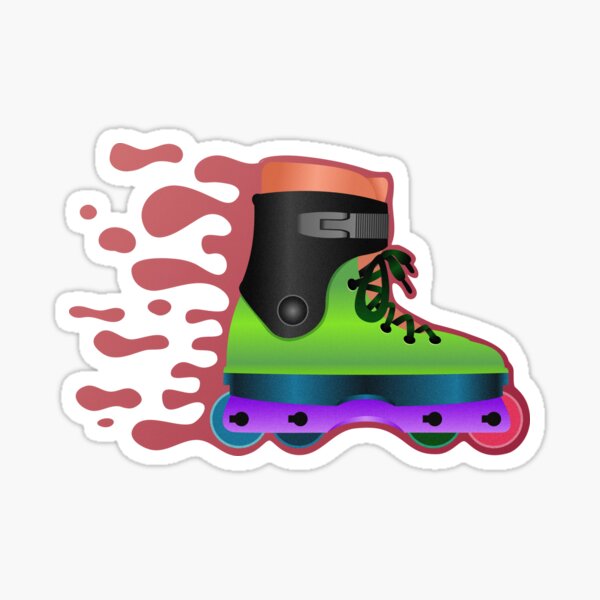The image is of a detailed sticker depicting a roller blade in motion, set against an off-white background with a white border and a silver outline. The roller blade is oriented to the right, showcasing a profile view. The boot's top portion is black with a gray strap, orange shin guards, and dark green laces. Its base is a vibrant neon green, and beneath that is a dark blue section followed by a bright purple rail. The four wheels, from left to right, are colored blue, dark blue, green, and pink. The inner sole of the boot appears to be peach-colored. The scene includes a darkish purple splash behind the boot, indicating movement, which some described as resembling wind or water splashes. The sticker is devoid of any text.